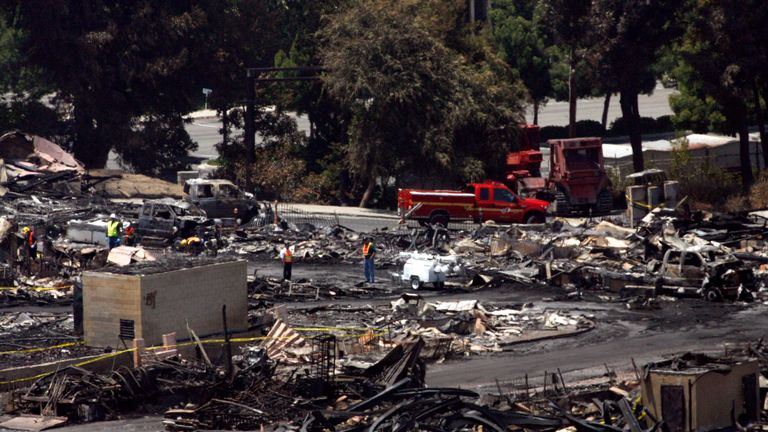This horizontally aligned rectangular image depicts the aftermath of a significant disaster, potentially a fire or a storm, at what appears to be a construction site or city dump. The foreground is littered with debris, including twisted metal, broken concrete, and a burnt-out car, creating what can only be described as a vast garbage field. Among the wreckage, several construction workers clad in bright orange and yellow safety vests with white hard hats can be seen, some standing idly, others seemingly assessing the scene.

A snaking road weaves through the debris, beginning on the left and curving in a U-turn before disappearing out of the frame on the right. In the middle of this chaotic landscape stands a low, rectangular concrete building surrounded by caution tape. Nearby, a red extended cab pickup truck with a yellow stripe, likely an emergency fire service vehicle, hints at the recent devastation. The background features a dense area of tall trees, their high branches forming a canopy over the scene. Beyond the trees, a parking lot and an unobstructed road are visible, contrasting starkly with the destruction in the foreground. This image captures a poignant moment of recovery amidst the remnants of a catastrophe.